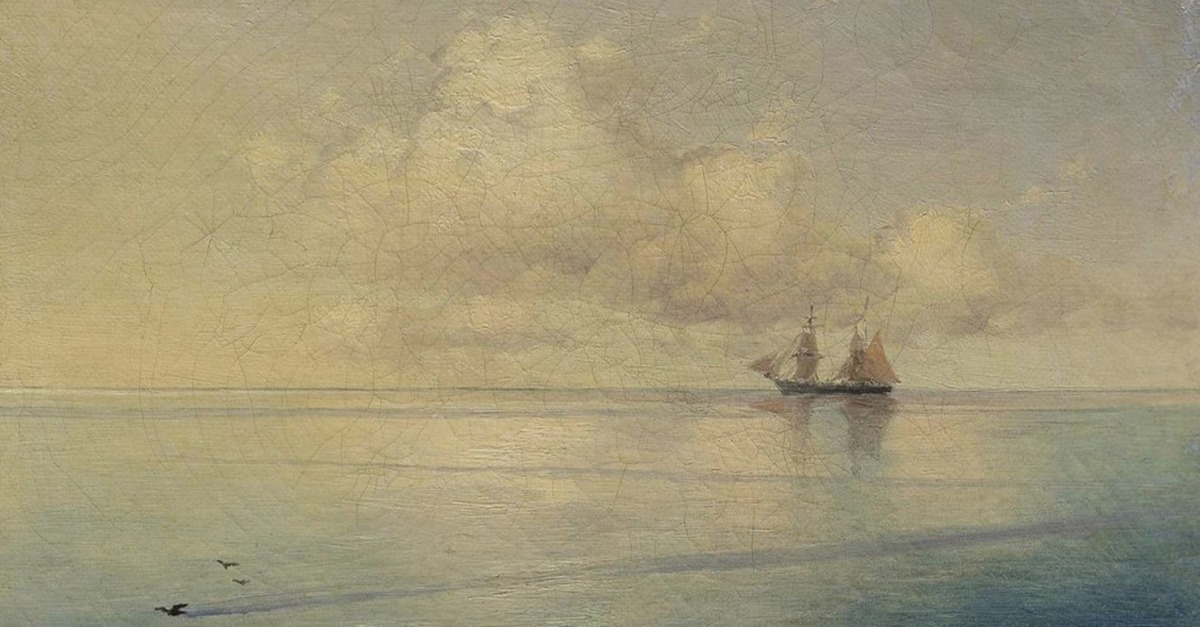The image is a detailed photograph of a slightly deteriorated oil painting, showing visible cracks and light brown lines across its surface. The scene depicts a serene outdoor setting, dominated by a calm, pale blue body of water, stretching toward the horizon. Positioned prominently in the distance is a large, 17th or 18th-century style ship with multiple masts and cream-colored sails, rendered in shades of black. Above the ship, the sky is adorned with gray and white clouds tinged with a hint of light purple. In the bottom left corner of the painting, three birds can be seen gracefully flying over the water's surface. The overall color scheme of the image features cool tones of blues and grays, creating a tranquil and slightly melancholic atmosphere.